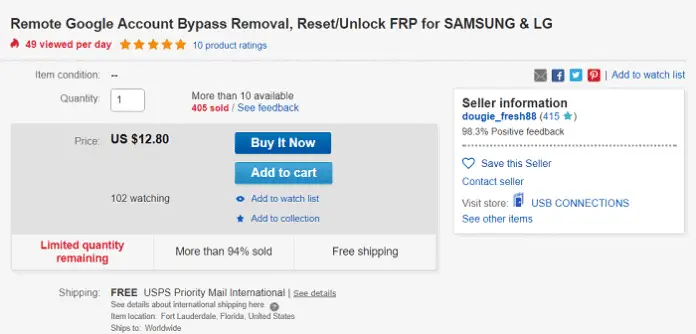A screenshot from a website, likely an e-commerce platform such as eBay although the site name is not visible, depicts a product listing with a light gray background and predominantly black font. To highlight specific elements, certain words are displayed in red, blue, and white fonts against various buttons and backgrounds for better contrast.

At the top of the screen, the product name is prominently displayed: "Remote Google Account Bypass Removal, Reset/Unlock FRP for Samsung and LG." Indicating its popularity, a flame icon is present to the left of the product name. Highlighted in red next to this icon, "49 viewed per day" signifies the high interest in this listing. In close proximity, a five-star rating is visible alongside a blue link indicating "10 product ratings."

Further down the page, various details about the product are provided:
- Condition of the item
- Available quantity
- Price
- Number of people watching the item

The urgency of the purchase is emphasized with red text proclaiming "Limited quantity remaining" and "More than 94% sold." The listing also mentions that the item comes with "Free USPS Priority Mail International" shipping.

On the right-hand side of the listing, seller information is prominently displayed, including their positive feedback rating and options to:
- Save the seller
- Contact the seller
- Visit the seller's store

Above the seller information, additional interactions are facilitated with options to email the listing, share it via Facebook, Twitter, or Pinterest, or add it to your watch list.